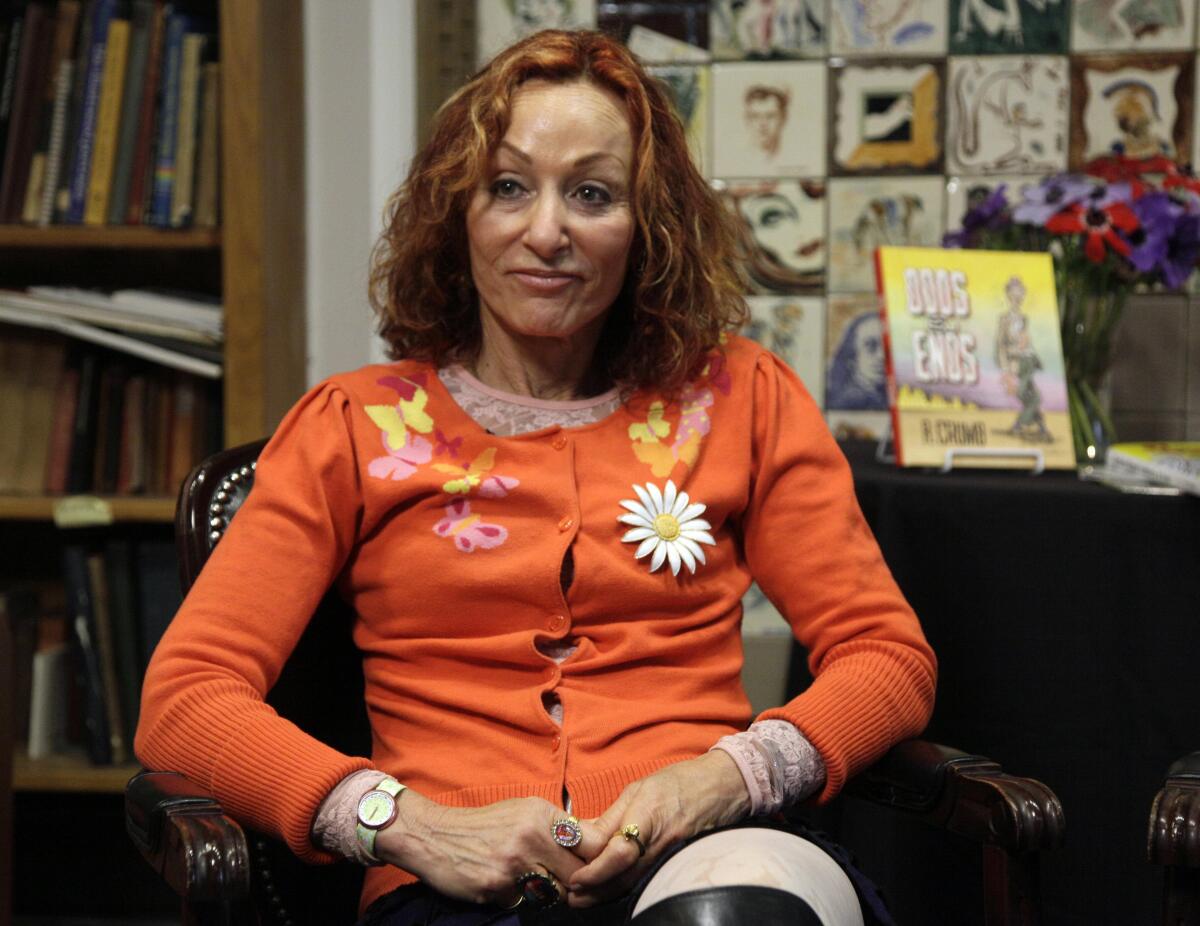A photograph captures a middle-aged woman with shoulder-length red hair adorned with golden highlights, sitting in a black leather chair. She appears to be in her late 40s or 50s, with a light complexion and warm brown eyes. Wearing a vibrant orange sweater decorated with a butterfly pattern—featuring yellow, pink, and purple butterflies—she pairs it with a pink lacy long-sleeved undershirt. On the right side of her chest, a white flower corsage with a yellow center adds a charming touch.

She accessorizes with a white watch on her left wrist, a red ring with a silver setting, a small golden ring on her right hand, and a few other rings on both hands. Her attire is completed with tall black boots and a short black skirt. The woman's eyebrows are slightly raised, and she sports a small, pleasant smile as she gazes at someone behind the camera.

The setting appears to be a cozy bookstore. Behind her, a wooden shelf filled with books is slightly blurred, creating a soft background ambiance. To the woman's immediate left and right, the walls are adorned with an eclectic mix of colorful and artistic pictures. On the desk beside her, a single book stands upright next to a vase filled with red and purple flowers. The book's title, "Gods and Ends" by R. Crumb, is partially readable, hinting at the surroundings rich with literary and artistic elements.